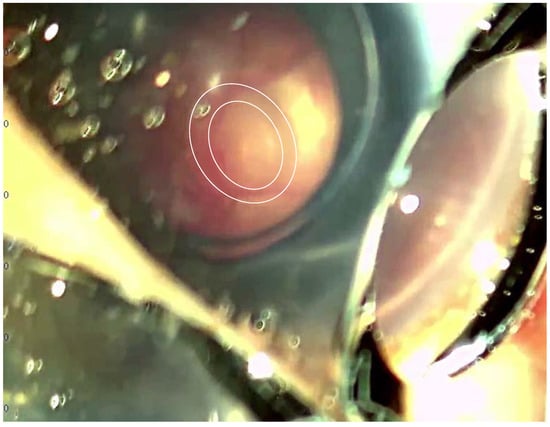This landscape-oriented image captures a close-up view that appears to be behind a blurry glass surface, reminiscent of looking through eyeglasses. In the center, there are two white ovals, one within the other, creating a distinct focal point. Surrounding this central feature are numerous circular shapes that resemble bubbles, with some appearing bright white and others having a greenish tint. To the right of the central ovals, there's a bright white light encircled by a black rim, evoking the appearance of an eyeglass lens or possibly part of a medical or surgical instrument. On the left, a yellow funnel shape descends towards the center, where it meets a solid white blotch at the bottom edge. Throughout the image, scattered white spots add to the overall impression of viewing through a fuzzy, reflective surface.